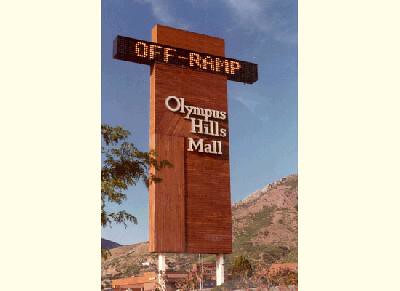This outdoor photograph captures a large, rectangular, reddish-brown wooden sign for Olympus Hills Mall, mounted on two white posts. The sign features a digital screen at the top, displaying the word "Off-ramp" in lit-up letters. Behind the sign, a stunning blue sky with wispy white clouds stretches across the background, while a dark-colored mountain and a green-brown grassy hill provide a scenic backdrop. To the left of the sign, the leafy branches of a tree partially extend into the frame. The detailed sign stands prominently against the natural landscape, creating a harmonious balance between natural and man-made elements.